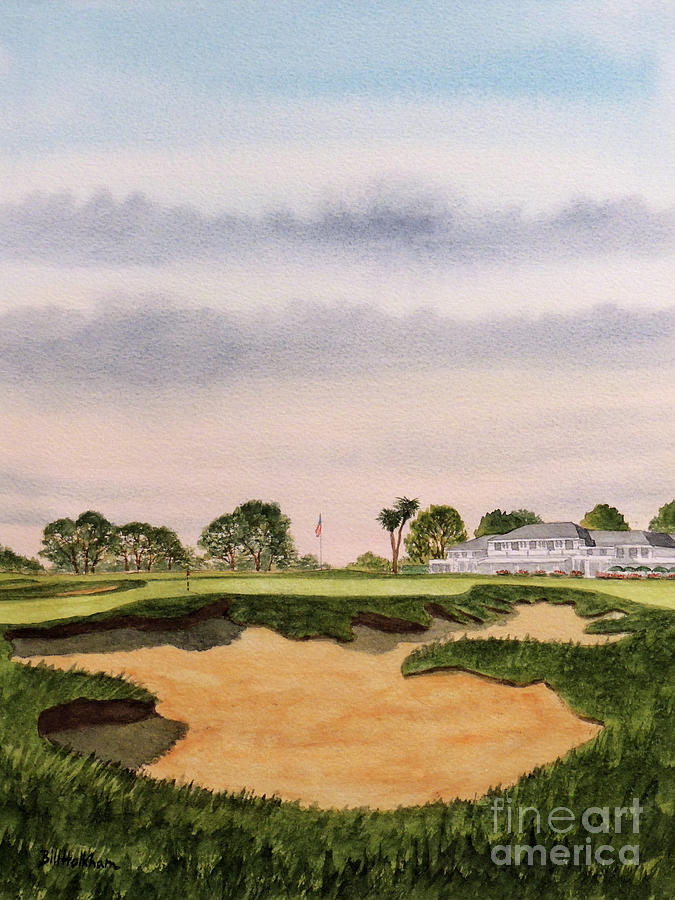The image depicts a finely detailed painting of a vast golf course under an overcast sky with shades of blue, white, gray, and hints of pink. The meticulously manicured green stretches across the canvas, interspersed with sandy dunes and various levels that give it a dynamic layout. Prominent in the scene is a large white building, possibly a clubhouse or a community center, situated to the right, with golf carts and cars parked nearby. The expansive field features multiple flags marking different parts of the course, and a brown patch of land contrasts against the lush greenery. Trees line the background, adding depth to the scene, while an American flag waves subtly in the middle distance. The painting is marked with the watermark "Fine Art America" in the bottom right corner.